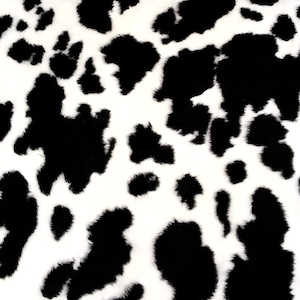The image is a black and white print featuring an abstract pattern of various black shapes set against a predominantly white background. The black shapes are irregular and scattered throughout the image, reminiscent of patterns found on a cowhide or a Dalmatian's fur. These shapes range from long and curvy to small and pointy, with no perfectly round circles. Several large black patches are located at the center, top, and bottom of the image. In particular, there are notable shapes—a large blob in the middle upper area that vaguely resembles the continent of Africa, another blob below it resembling an animal with humps and four legs, and an oblong shape curving to the right at the bottom. Other discernible shapes include one that resembles a rabbit, another that looks like a rhinoceros, a mermaid-like figure, and a head of a dog protruding from a pedestal. The textured blending of black and white suggests the appearance of fur, adding to the impression of cowhide.